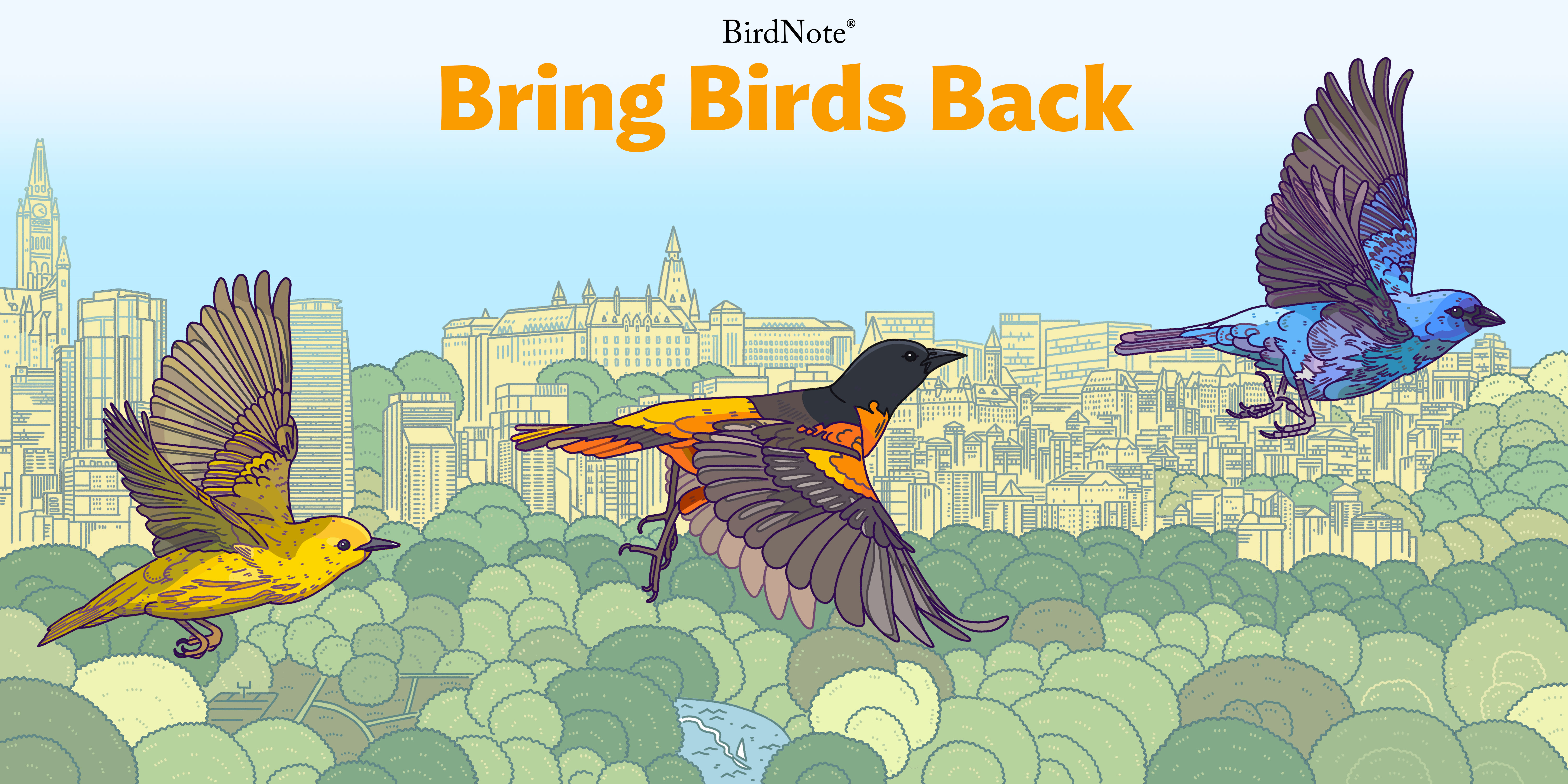A vibrant, cartoon-like digital drawing titled "Bird Note: Bring Birds Back" features three small, exotic birds in flight against a backdrop of a thriving downtown area, possibly New York City. The birds—illustrated in smooth, pastel shades—ascend in a diagonal formation above a lush canopy of trees, reminiscent of Central Park. The leading bird is predominantly blue with hints of gray, followed by a middle bird with an orange body and a black head, while the trailing bird is a striking yellow with brown accents. The background boasts towering skyscrapers rendered in muted beige tones, under a light blue gradient sky. Below the birds, a serene river with a sailboat and a farming field add depth to the scene, emphasizing the contrast between the urban and natural environments. The artwork seems to advocate for environmental conservation, aiming to raise awareness about the decline in bird populations and the need to restore their habitats.